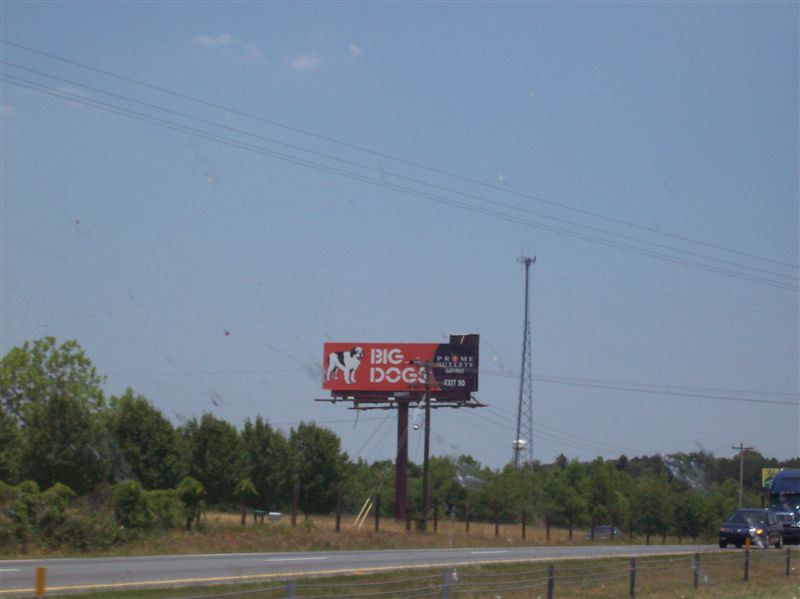In the foreground of the image, there is a street visible at the very bottom. Off in the distance on the right side of the image, a car is driving towards the observer, with a partial view of a large semi-truck following behind it. The background is filled with a dense cluster of deciduous trees. 

Dominating the middle of the image is a very tall pole supporting a bright red billboard. The billboard prominently features the text "Big Dogs" and includes an image on the left of a white dog with black spots. To the right of the dog image, there is a black field with text that is too small to read. In the far distance, a transmission tower can be seen along with electrical lines crisscrossing through the frame, adding layers of visual complexity to the scene.